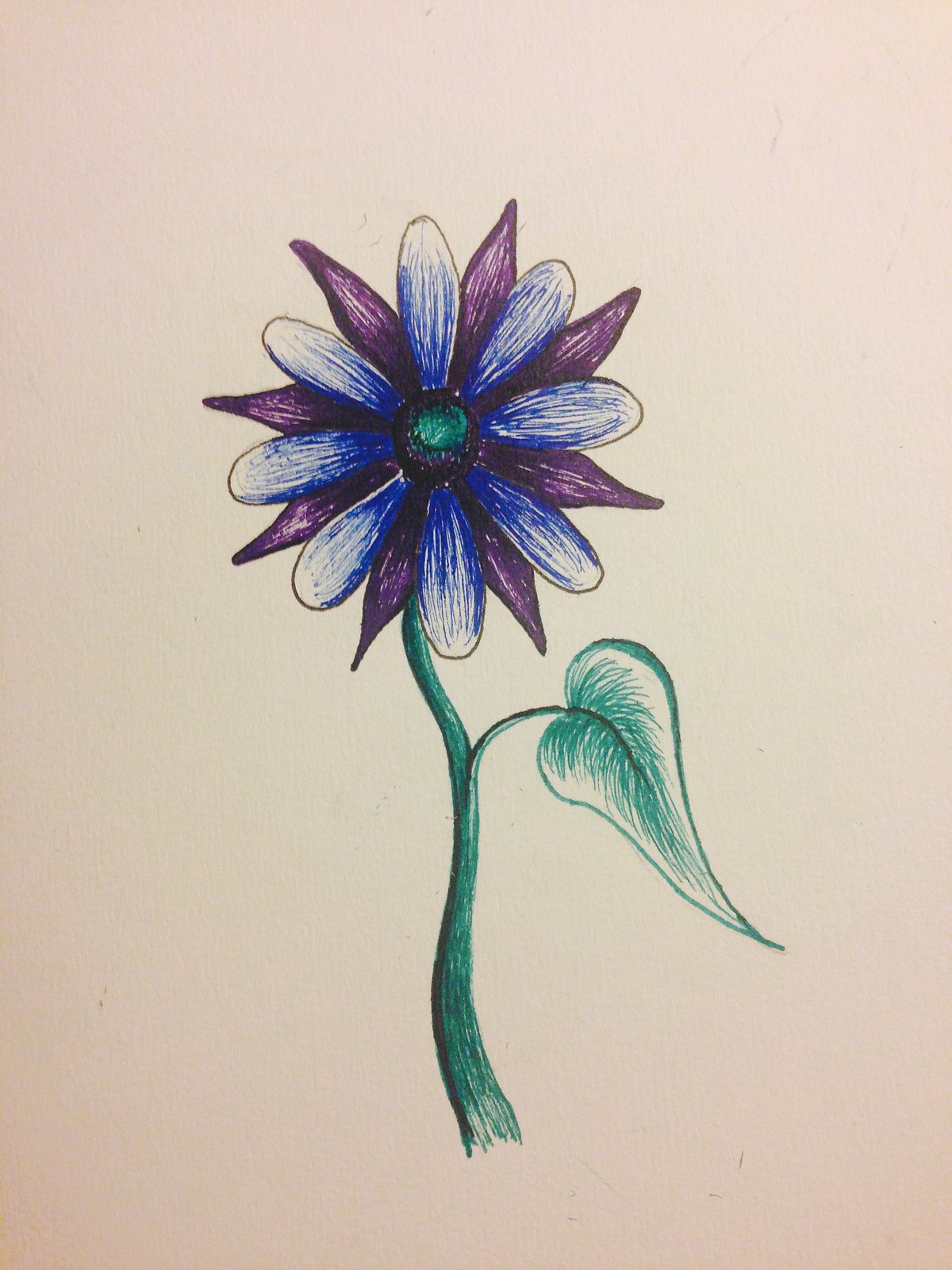In this zoomed-in image of a drawing on white paper, the confines of the paper and the surface it rests on are not visible. The artwork features a delicate flower created with green, black, blue, and violet-purplish colored pencils. A gently curving green stem, interspersed with black lines for texture, extends upwards and is adorned with a heart-shaped leaf. At the top of the stem, a flower blooms with two distinct sets of petals: the top set consists of blue, oval-shaped petals, while the set beneath features pointed, violet-purple petals. The perspective of the drawing suggests a view from above, highlighting the intricate details and vibrant hues of the flower.